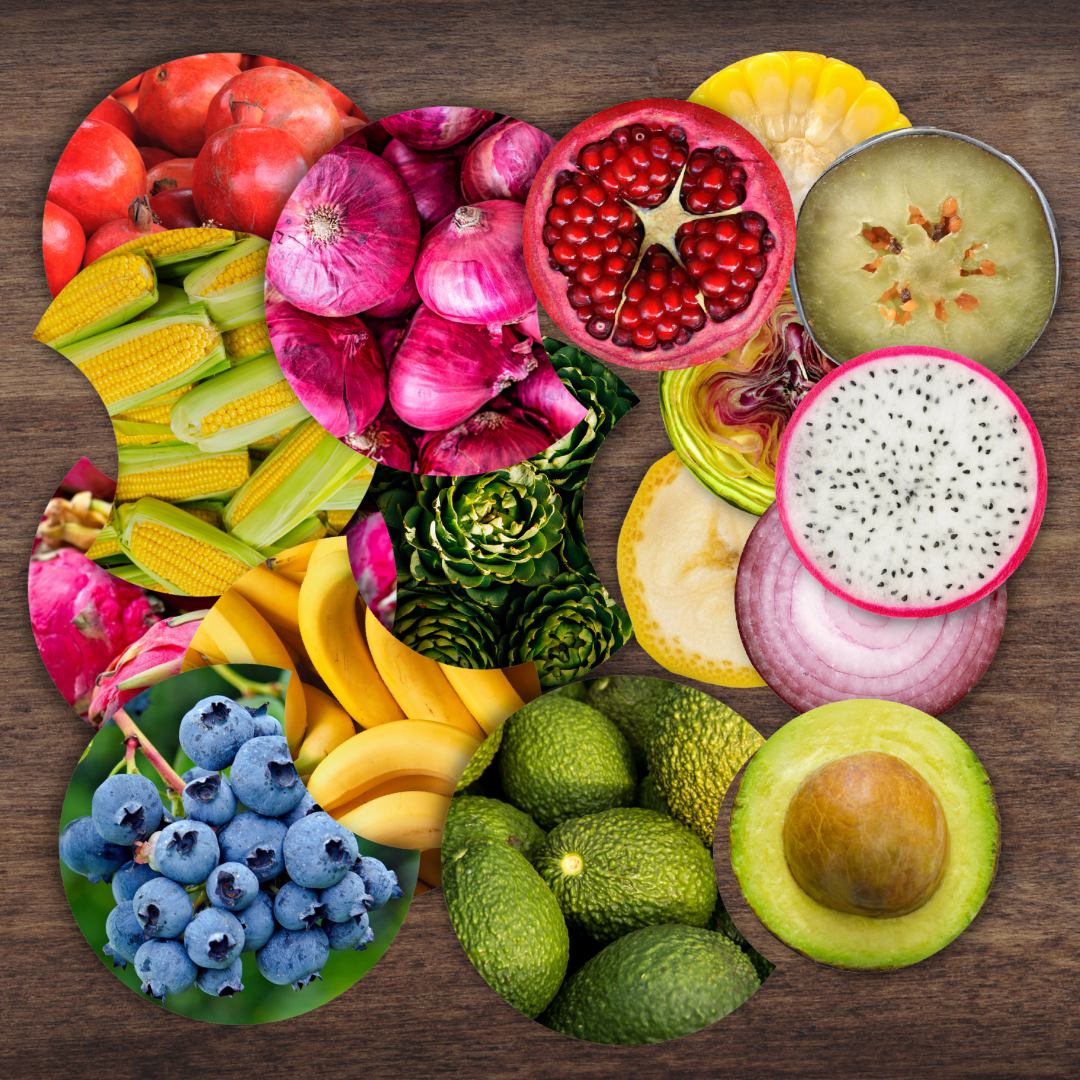This is a digital collage of various fruits and vegetables, meticulously arranged in an overlapping, circular pattern and set against a dark brown, wooden texture background. The collage features vibrant and richly colored produce, including red onions, pomegranates, dragon fruit, corn, bananas, blueberries, avocados, and tomatoes. Some circular cutouts have bites taken out, resembling a partially eclipsed moon. The images are erratically yet artistically overlaid, providing a dynamic and visually engaging composition. The fruits and vegetables are depicted in diverse stages, such as whole, sliced, and even with a section missing, adding complexity to the display.